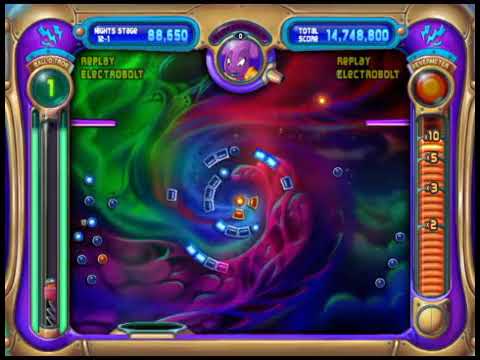This image is a screenshot from a video game set in outer space, featuring an intricate display of swirling galaxy clouds in vibrant colors of green, purple, blue, red, and pink. The center of the screen showcases a vortex that draws in four rounded rectangle shapes, resembling bricks that are blue and gray, with some containing orange centers and dots. These floating shapes are part of a captivating, mystical swirl pattern with additional glowing blue and orange dots circling around.

Framing the game screen is a rounded golden rectangle. The left vertical border houses a meter with a purple background, a green circle labeled "1" at the top, and illuminated green bars at the bottom. The right vertical border has an orange scale marked with increments of 2, 3, 5, and 10; the meter is nearly maxed out to the "times 10" mark. At the upper left and right corners, the text "Replay, Electro Bolt" is visible. The top of the screen displays a score, with one number reading 88,650 and another indicating a total score of 14,748,800. Dominating the upper center of the screen is a character encapsulated in a circle, purple in color, reminiscent of a Pokémon-style character.